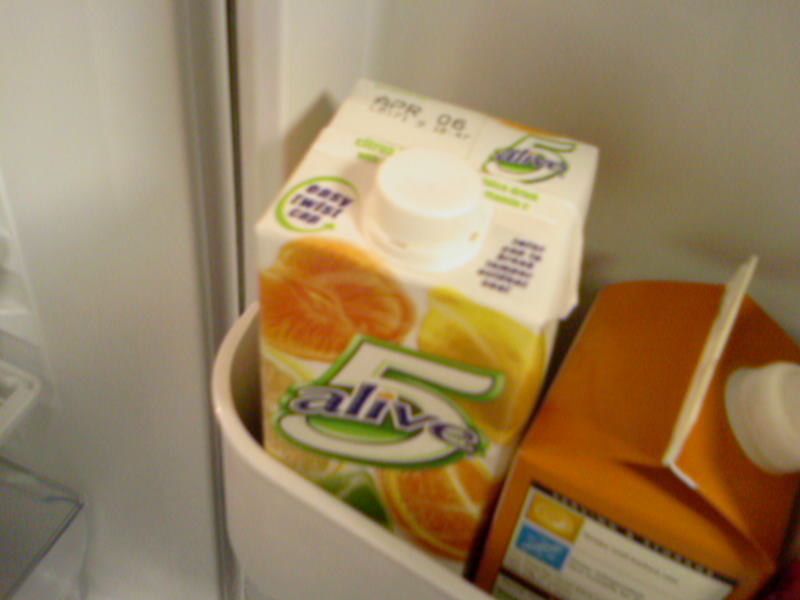The image showcases the interior of a refrigerator door, focusing on one of its shelves. Prominently displayed on this shelf is an unopened carton of Five Alive citrus beverage, identifiable by its white packaging bordered with green and adorned with the word "alive" in lowercase blue letters, with the dot on the "i" in orange. This particular carton, designed to resemble a traditional milk container, advertises a blend of five citrus juices and has a printed expiration date of April 06. Positioned beside it is a more conventional orange juice carton with a pointed top and a white label. Additionally, the image offers a glimpse of adjacent refrigerator components, including the crispers and other shelves, visible towards the left, near the door hinge area.